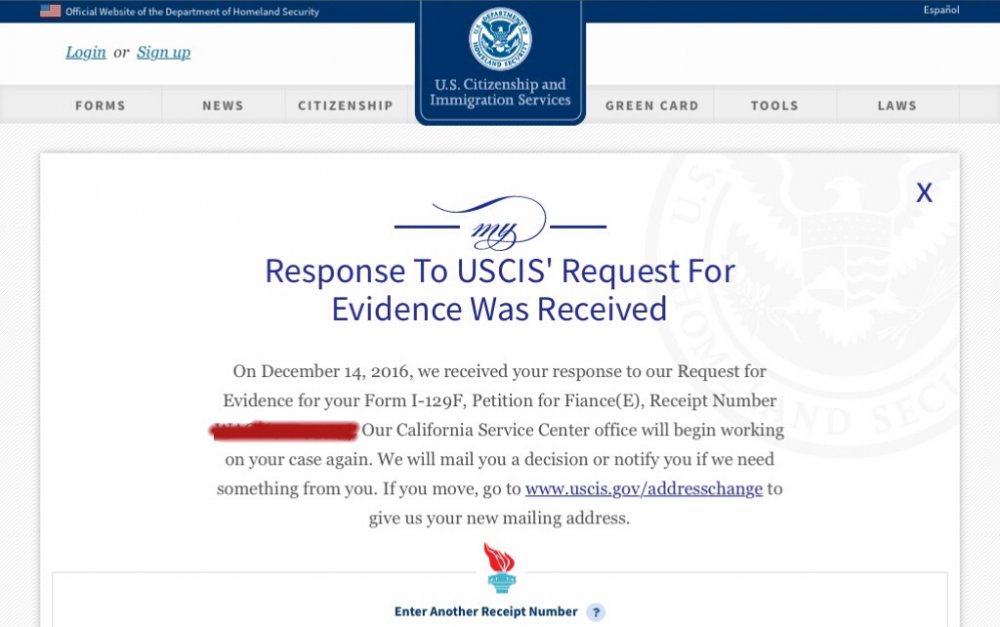The image shows a screenshot of a webpage with a white background, featuring the official seal at the top. The header indicates that this is a page from the U.S. Citizenship and Immigration Services (USCIS) website. In the top right corner, there is an option to switch the language to Español. Below the header, there are various navigation links labeled "Login or Sign Up," "Forms," "News," "Citizenship," "Green Card," "Tools," and "Laws."

The main body of the page contains a notification regarding a user's response to a USCIS request for evidence (RFE). The message reads: "On December 14, 2016, we received your response to our request for evidence for your Form I-129F, Petition for Alien Fiancé(e), receipt number (blocked out in red). Our California Service Center office will begin working on your case again. We will mail you a decision or notify you if we need something further. If you move, please go to www.uscis.gov/addresschange to update your mailing address."